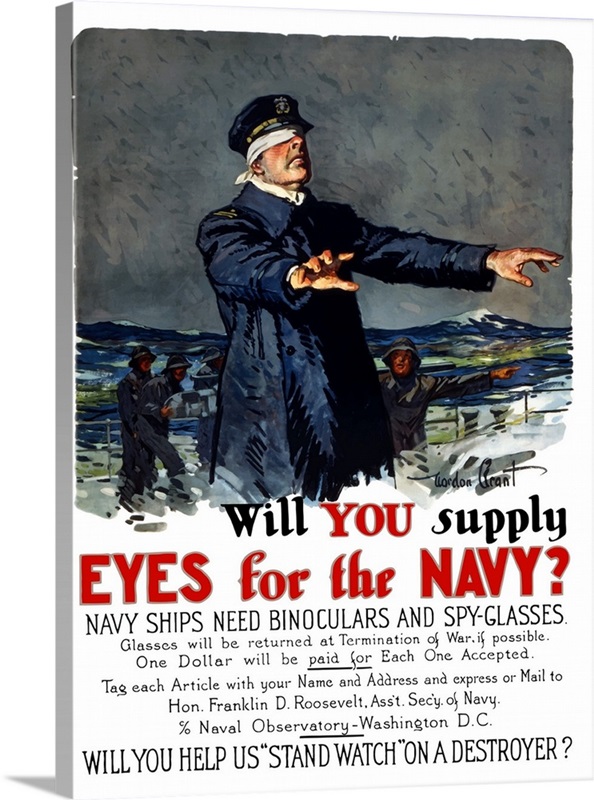The image is a reproduction of an old World War I poster, featuring a detailed painting of a naval officer. The poster is in a rectangular portrait format, with approximately the top 60% dedicated to the illustration. At the forefront, a man in a blue navy uniform, including a heavy overcoat and a cap, is depicted wearing a white blindfold. His arms are outstretched in front of him, as if seeking something, with his hands visible from his coat sleeves. Behind him, three smaller figures, appearing to be seamen in gray jackets and navy hats, operate equipment. One seaman points to the right, while the others face the viewer. They are positioned on what seems to be the deck of a ship, with a railing and a rocky sea illustrated in the background under a stormy, gray sky. 

The bottom half of the poster consists of text in bold, black and red fonts, urging, "WILL YOU SUPPLY EYES FOR THE NAVY?" The following smaller text explains, "Naval ships need binoculars and spy glasses. Glasses will be returned at termination of war if possible. One dollar will be paid for each one accepted. Tag each article with your name and address and express or mail to Hon. Franklin D. Roosevelt, Assistant Secretary of the Navy, Navy Department, Washington, D.C." The poster concludes with the phrase "WILL YOU HELP US STAND WATCH ON A DESTROYER?" emphasizing the call to action. The artist's signature, partially legible, can be found in the bottom right corner of the image.